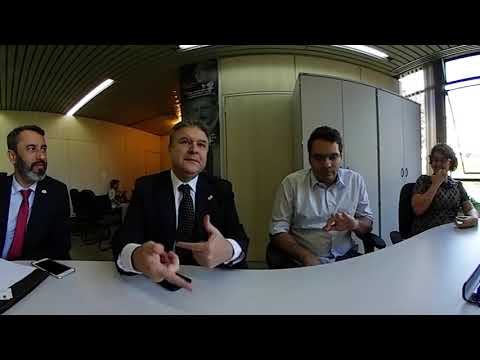In the image, four people are seated at a light blue-colored, slightly curved table inside a room. The two men on the left are both dressed in black suits and ties. The man furthest left is looking at the man next to him, who has his right arm extended forward and fingers pointed in different directions, seemingly making a point. A cell phone and some documents are placed in front of them. Just next to the man making a point, there’s another man wearing a white shirt with his sleeves rolled up, looking down. To the right of him sits a woman with short gray hair, wearing a brown dress or blouse, and holding a finger to her mouth. The setting includes a beige and brown ceiling, beige walls, and fluorescent lights. Behind the group, there’s a curved, bubbly cabinet, and to the right, an open window along with light gray lockers. There are also a few other individuals seen sitting in the background.